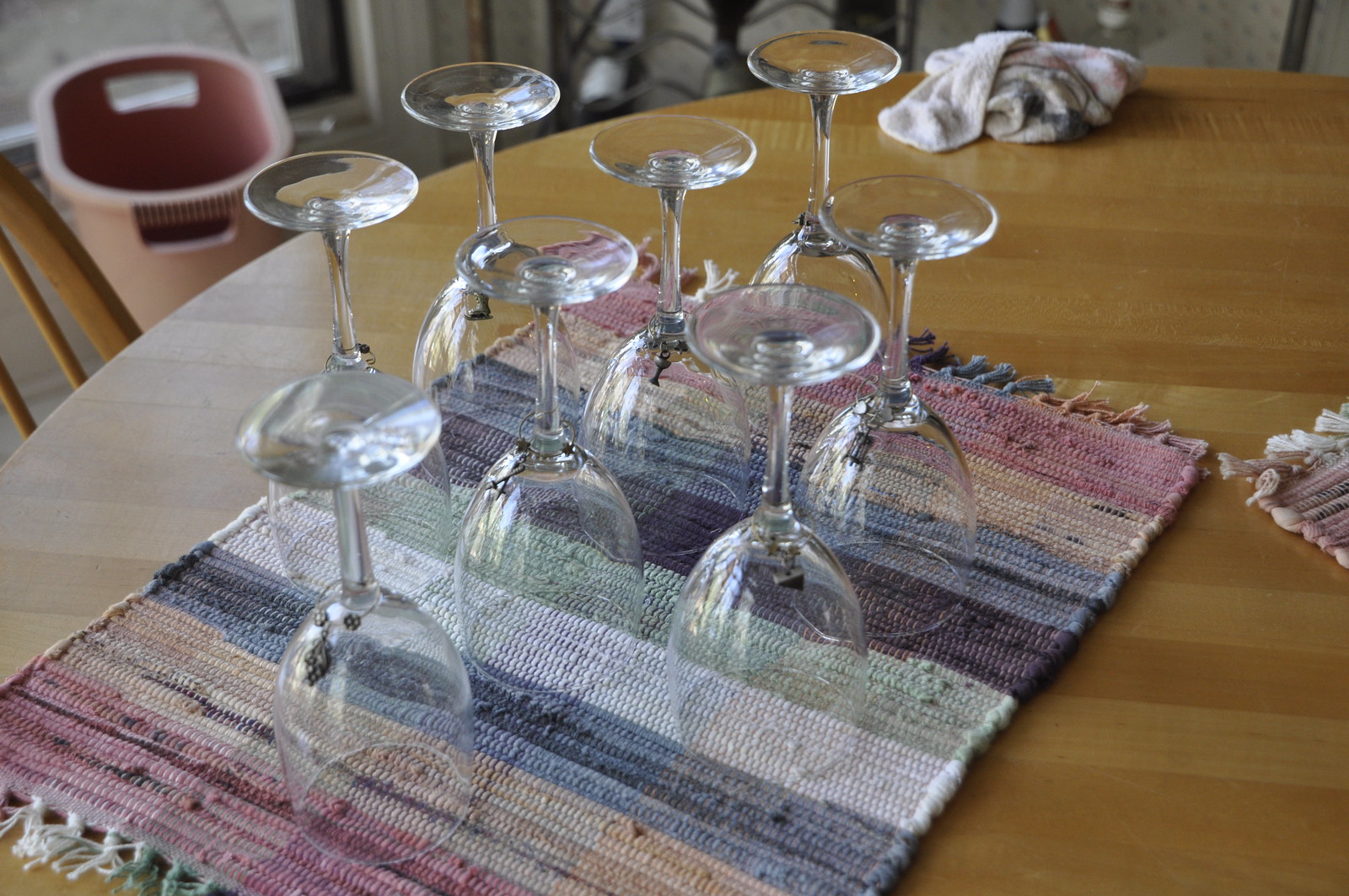In the image, a round dining room table made of blonde wood features prominently. Atop the table lies a vibrant woven placemat adorned with vertical stripes in muted shades of pink, green, blue, and orange, with fringes at both ends. This placemat hosts eight medium-sized, clear wine glasses, each placed upside down to dry. Beside the placemat, part of another striped cloth is visible, along with a white rag haphazardly tossed near the edge of the table. In the background, to the upper left, a pink trash can sits in front of a window, and a wooden chair with a slatted back peeks into the frame, adding depth to the scene. The image is devoid of any text or words.